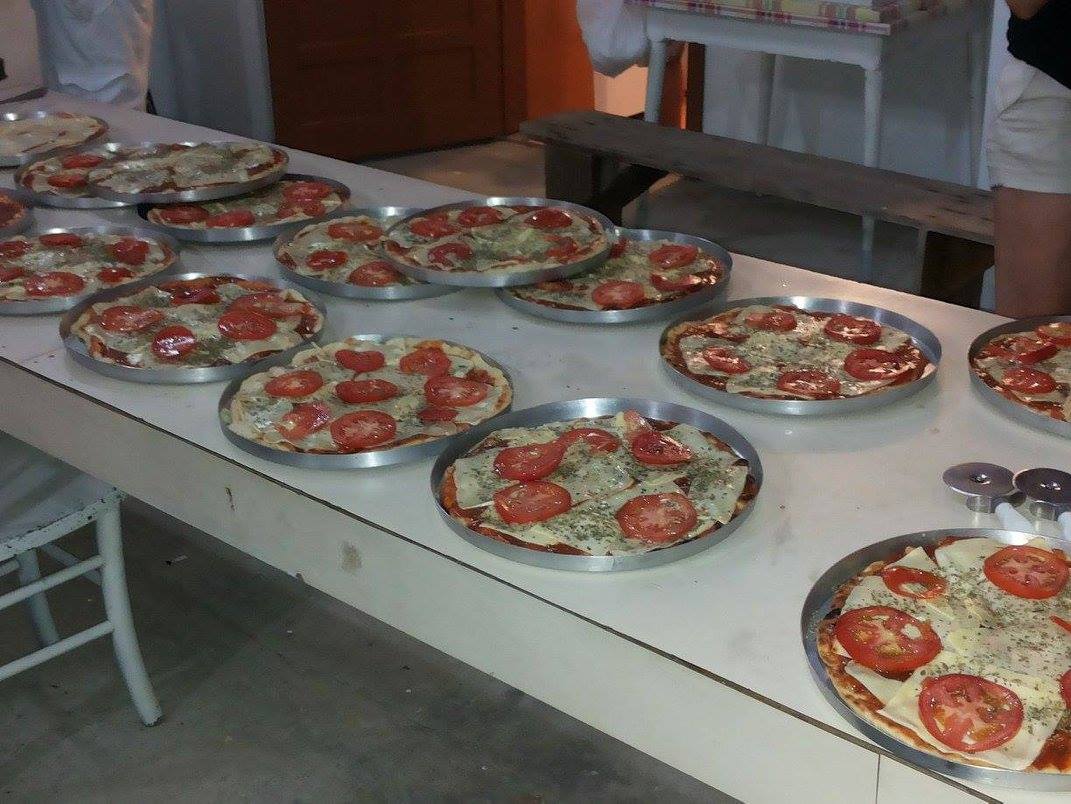The image depicts a set of approximately 14-15 circular metal plates, each holding what appears to be an uncooked margherita pizza, arranged on a long, white table. The pizzas are laid out in a line, with some slightly overlapping each other. Each pizza is composed of a round, dough base topped with tomato sauce, square slices of white cheese, and sliced tomatoes, adorned with dried herbs, likely basil or similar spices. The white table, which is a couple of inches thick, is situated above a white chair with grey stripes and near a wooden bench. The setting appears to be a preparation area, possibly in a restaurant or event space, as glimpses of people in white outfits and shorts can be seen working in the background on what looks like a cement floor.